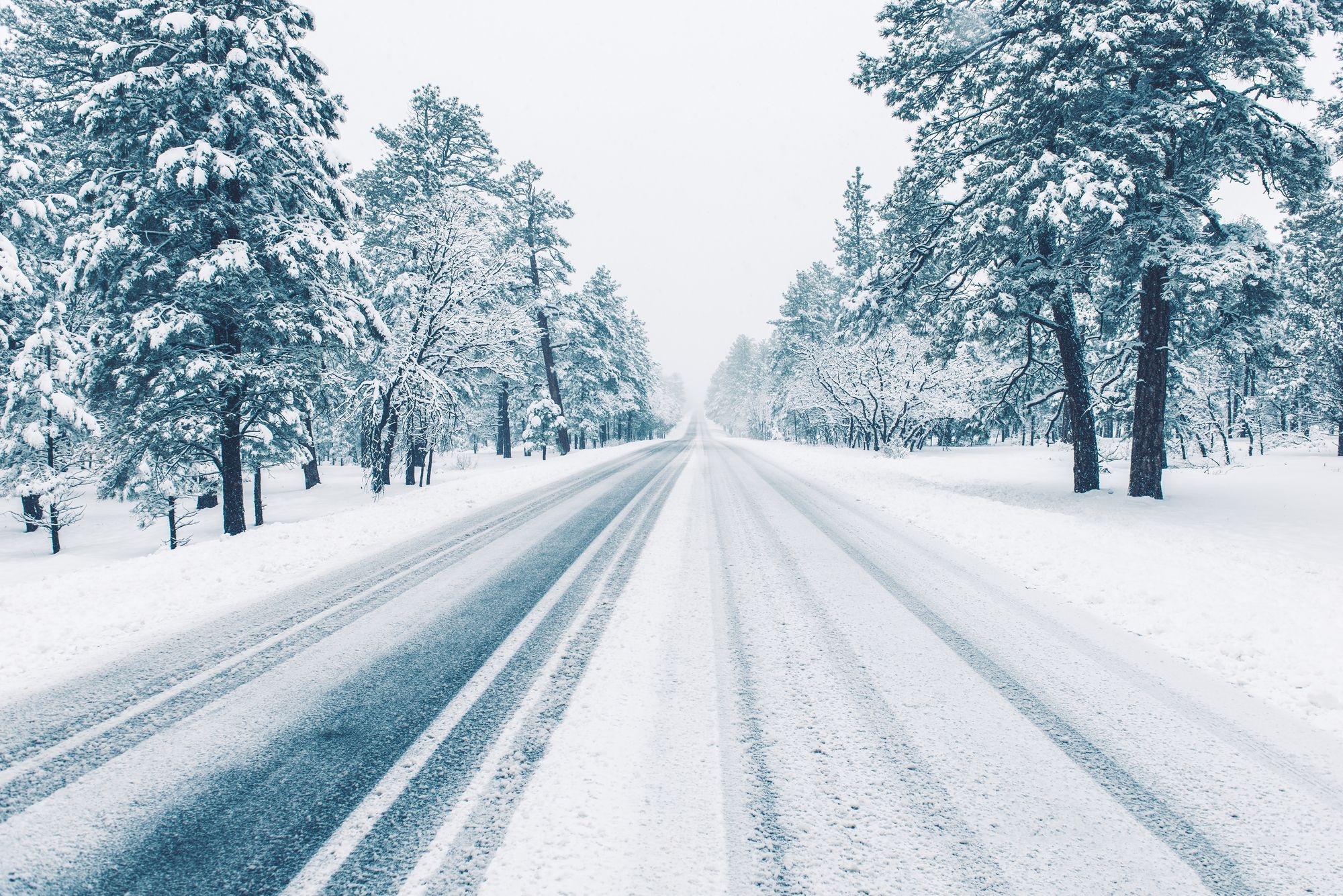This is a photograph capturing a serene, snowy day on a deserted highway. The road, covered with a thick blanket of snow, is only visible through dark tire tracks that create a striking contrast against the white expanse. These tracks, slightly melting the snow beneath them, depict the passage of previous traffic. Surrounding the highway on both sides are dense arrangements of evergreen and pine trees, their branches heavily laden with glistening clumps of snow, some bending under the weight. The dark green foliage and almost black tree trunks contrast sharply with the pure white snow, adding depth and texture to the image. The backdrop features a muted, almost completely white sky that emphasizes the brightness of the scene and suggests an open, expansive distance. Overall, the photograph encapsulates the quiet beauty and stillness of a winter landscape, with its play of dark greens, whites, and the starkness of a snow-covered road stretching into the horizon.